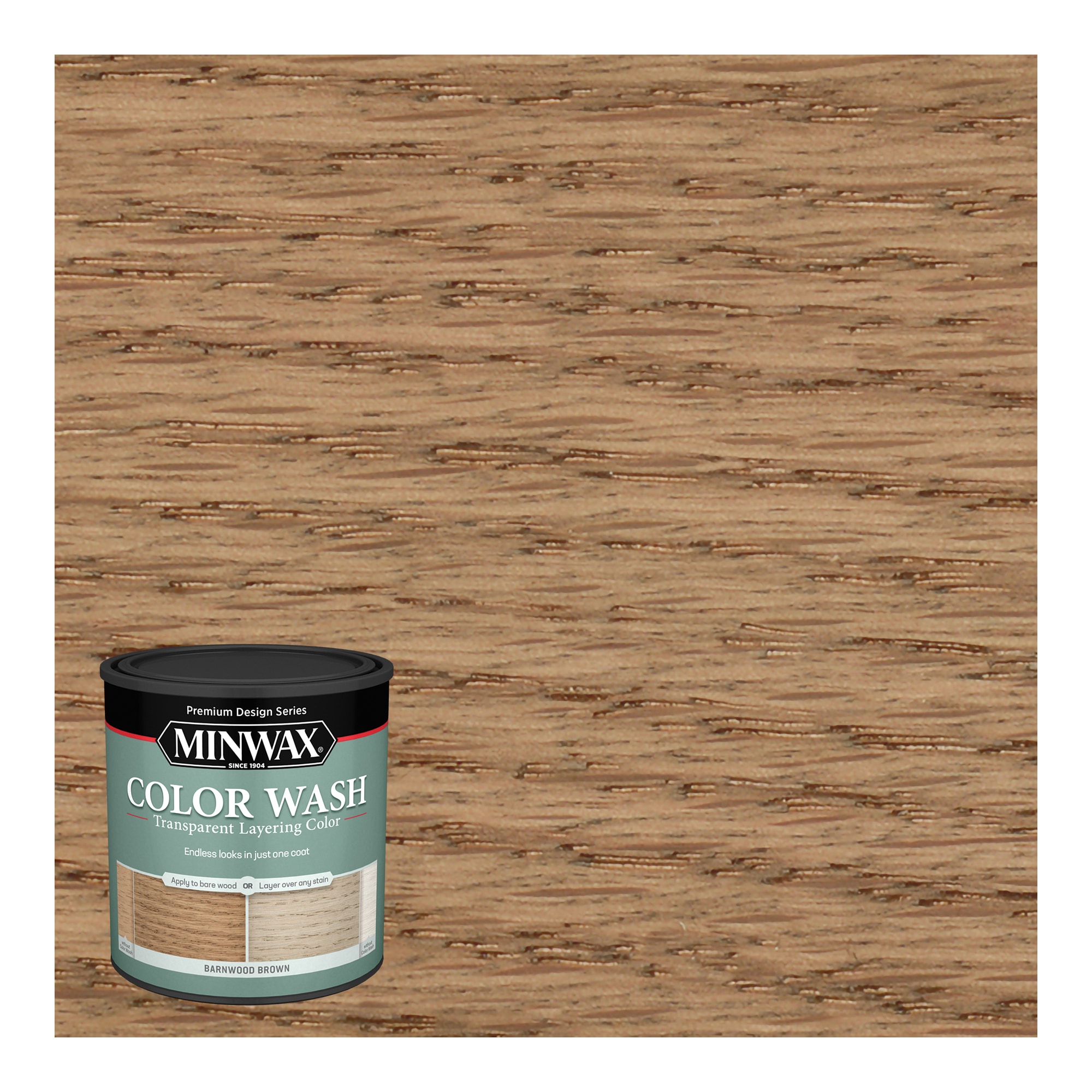The image captures a detailed view of a wooden surface that has been treated with a brown color wash, featuring a light beige base with darker brown streaks and spots running horizontally across the surface. In the bottom left corner, there is a prominently visible can of Minwax paint. The can is characterized by its dark gray lid and a black band just below the lid, with the inscription "Premium Design Series" in small letters. The larger white letters on the can read "Minwax," and beneath that, there's a light turquoise section with the words "Color Wash" in white, followed by "Transparent Layering Color" and "Endless Looks in Just One Coat." The bottom part of the can depicts two samples of wood finishes: one showcasing the described beige and brown streaked effect, and another presenting a primarily gray variation, indicating different possible effects achieved by the same product. The can also notes the color "Barnwood Brown" as the featured shade. The overall image is bright and clear, highlighting the texture and finish of the treated wood surface with precision.